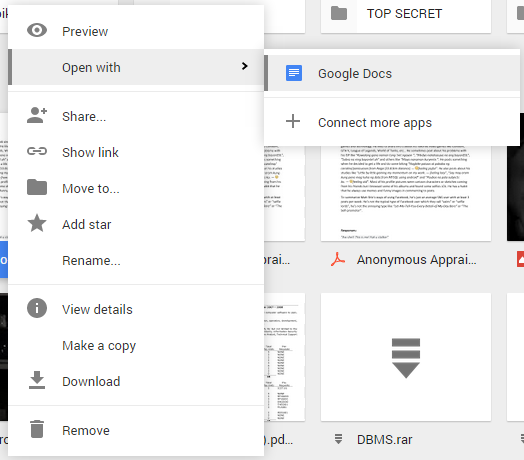The image depicts an individual interacting with a Google Drive interface. In the background, a grid of selectable documents is visible, arranged in a tile format. One particular document has been selected, and the user is currently viewing a dropdown menu of options. These options include: Preview, Open with, Share, Get link, Move to, Add star, Rename, View details, Make a copy, Download, and Remove.

The user has highlighted the "Open with" option, revealing Google Docs as the sole application currently available. Beneath Google Docs, there is a plus icon accompanied by the text "Connect more apps," indicating that additional applications can be connected for file opening.

In the background, various files can be discerned. Notably, one document is labeled "anonymous appray," likely intended to read "anonymous appraisal." Another file below it is named "dbms.rar." Prominently at the top of the background, a folder labeled "Top Secret" is visible. Although partially obscured by the dropdown menu, there are glimpses of other tiles with indistinct labels and colors, including a noticeable blue "O" to the left of the dropdown menu.

The majority of the screen background is an off-white color, contributing to a clean and organized appearance. The combination of the visible tiles, labels, and the detailed dropdown menu create a comprehensive depiction of a typical session of navigating and managing documents within Google Drive.